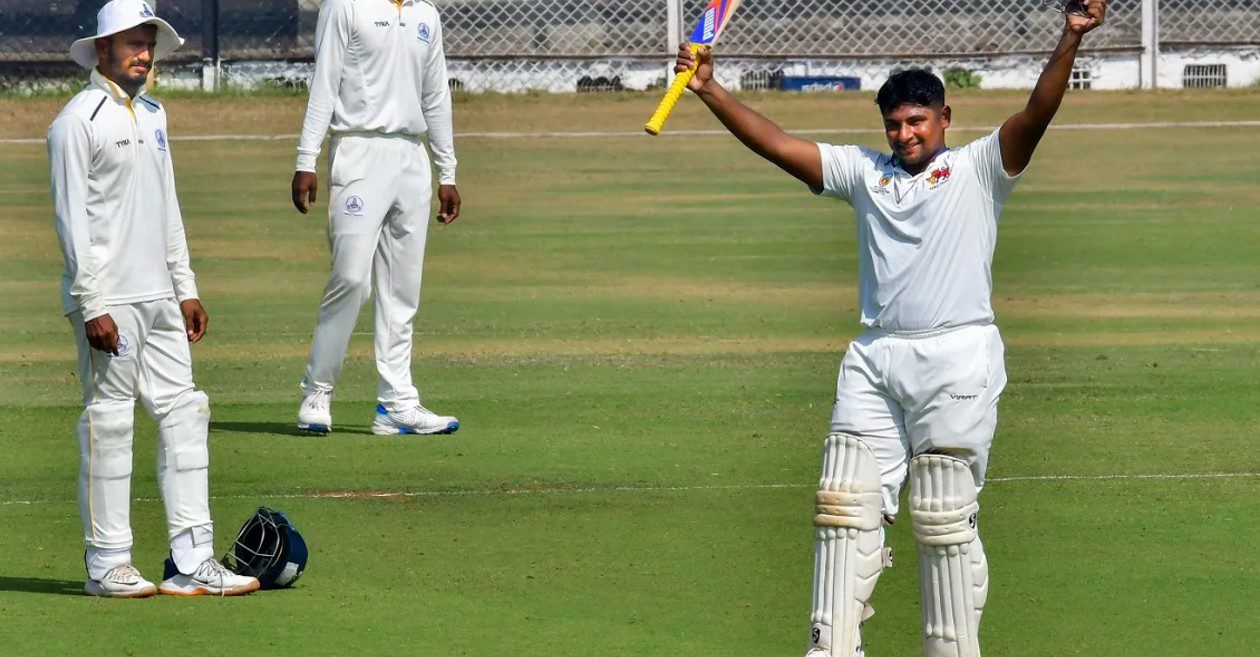In this horizontally oriented photograph, three individuals are standing on what appears to be a cricket field. The player on the right, who has a South Asian appearance, is dressed in a white t-shirt and white pants with protective padding visible beneath his attire. He jubilantly raises his hands, one of which holds a cricket bat, suggesting he has just scored. The other two players, dressed similarly in white shirts, long white trousers, and leg padding, share the scene. One of these players wears a black helmet and is seated on the grass. The expansive, lush, green field stretches out around them. The photograph shows the full bodies of the two players on the left, while the player on the right is partially cut off at the top, with his head extending beyond the photograph's border. The scene captures a moment of celebration on the cricket field.